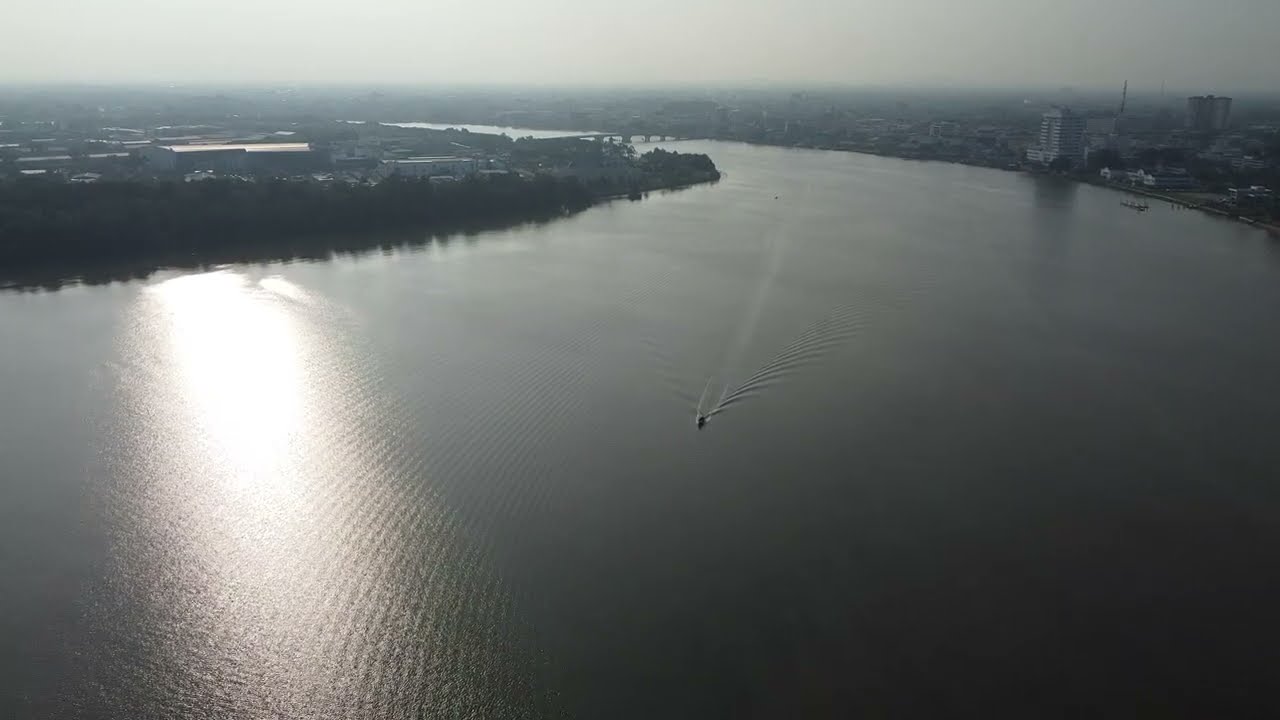This overhead photograph, captured by a drone or helicopter, depicts a large, meandering river on a foggy day. The sky is a milky gray, casting a soft, filtered light that reflects brightly off the water's surface on the left side of the image. The winding river flows from the upper left of the horizon towards the foreground, which is flat and straight, enhancing the natural landscape devoid of significant urban development. The serene water, which appears gray due to the fog, is subtly disturbed by the presence of a small motorboat or speedboat. The boat, positioned towards the center of the image, moves towards the foreground, leaving visible trails in the water. The surrounding area on both sides of the river features a few unremarkable buildings, possibly part of a modest town or city, though none are tall enough to be considered skyscrapers. A dense fog blankets the scene, further suggesting a serene Midwestern setting.